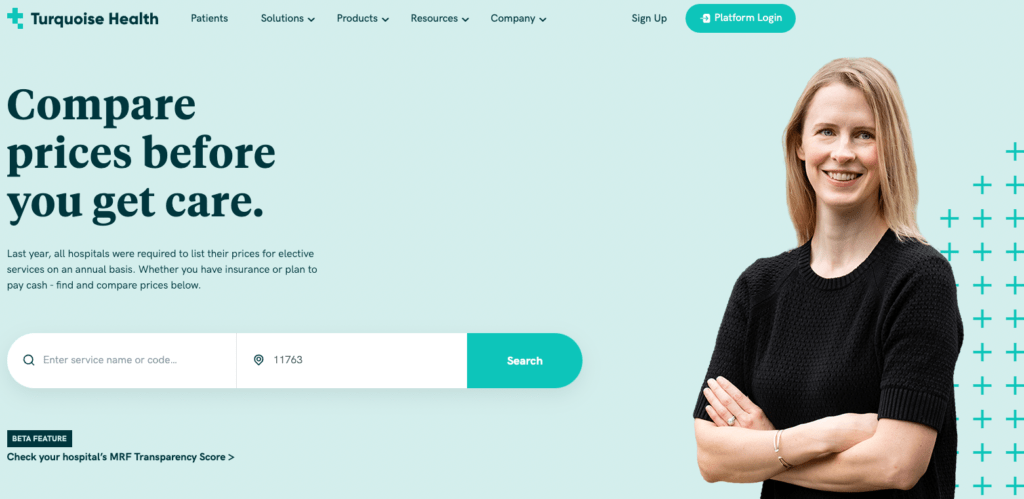This image is a screenshot of a website called Turquoise Health, characterized by a modern and clean design. 

**Top Section:**
- **Logo**: Positioned at the top left, featuring a medical plus sign with a small blue square at the bottom right. The plus sign is in a turquoise blue color. To the right of the symbol, "Turquoise Health" is written in dark blue text.
- **Navigation**: To the right of the logo, there is a navigation menu comprising:
  - Patients
  - Solutions (with a drop-down icon)
  - Products (with a drop-down icon)
  - Resources (with a drop-down icon)
  - Company (with a drop-down icon)
- **Sign-Up and Login**: Further to the right, there is an option for "Sign Up". Adjacent to it is a "Platform Login" button in turquoise color, rounded on both sides with white text.

**Hero Section:**
- **Background Color**: The section has a light sky blue-grayish hue.
- **Main Text**: The largest text in dark blue reads, "Compare Prices Before You Get Care." spread across three lines.
- **Subtext**: Below it, a paragraph explains, "Last year, all hospitals were required to list their prices for elective services on an annual basis. Whether you have insurance or plan to pay cash, find and compare prices below."
- **Search Bar**: Situated below the subtext, the search bar is large with rounded edges and consists of three sections:
  - A search icon followed by the placeholder text, "Enter Service Name or Code".
  - A location icon followed by the placeholder text, "11763".
  - A "Search" button in turquoise color with white letters.
  
**Beta Feature:** Below the search bar, inside a dark blue square with white text, the phrase "beta feature" is written. Beneath this, in blue letters, it reads, "Check Your Hospital's MRF Transparency Score Greater Than."

**Image Section:**
- To the right of the hero section, a photograph depicts a smiling woman with shoulder-length blonde or possibly red hair, wearing a black, short-sleeve knit sweater. She has her arms crossed over her chest, accessorized with a gold bracelet and a ring. Behind her is a design element featuring a pattern of plus signs.

Overall, the website's layout is methodically structured, balancing informative text with inviting visuals to enhance user engagement.